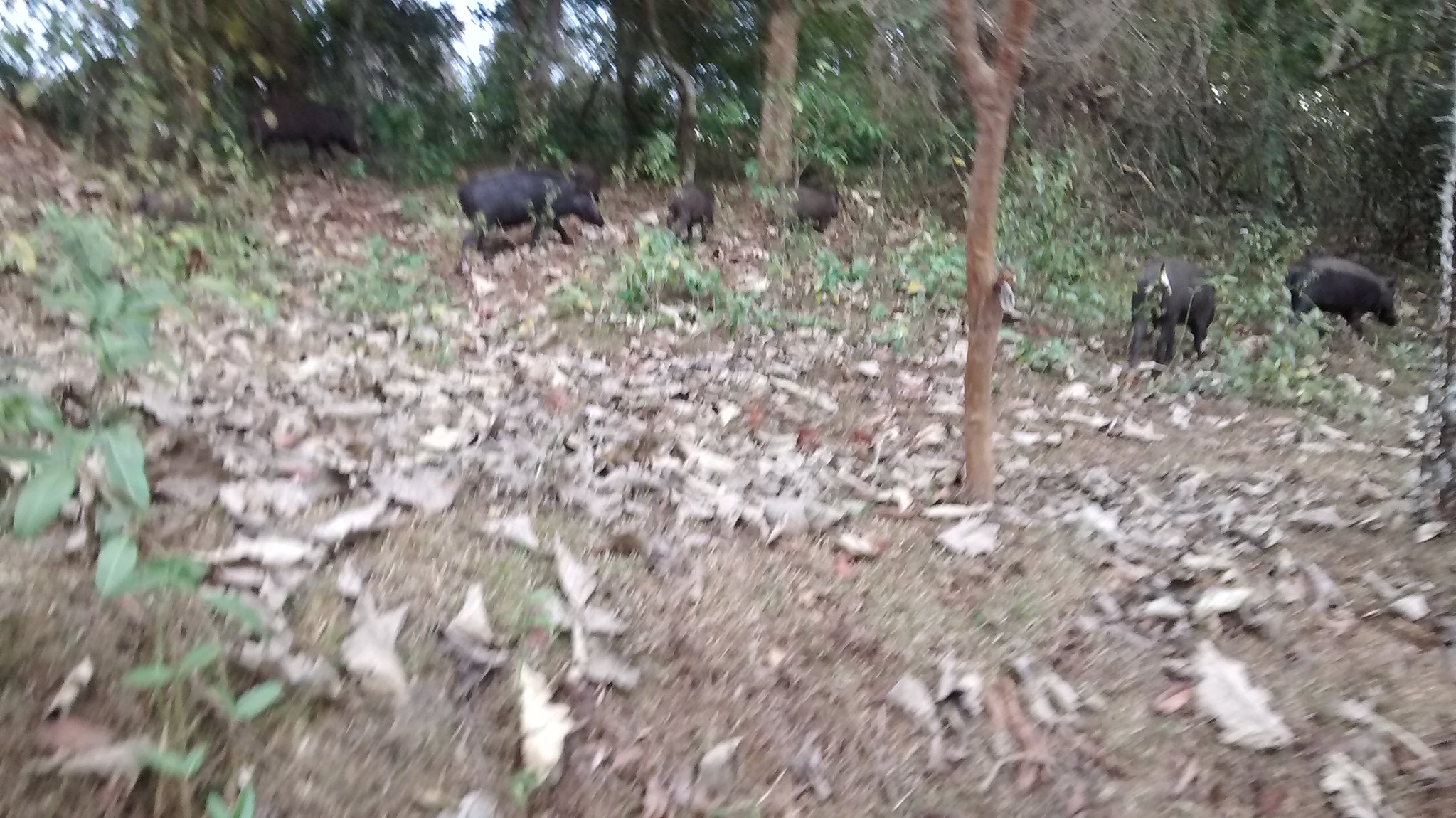This is a blurry photograph showcasing five wild boars in a wooded area. The boars, black in color, are scattered across a forest floor covered with dead leaves and brown, dying grass. Some patches of green and vines can be seen among the trees and blurry forestry in the background, with a hint of white sky peeking through. One tree stands towards the front of the picture, while another is situated towards the back. Among the animals, three boars are aligned, walking along a path towards the back of the image, and two are on the right-hand side, with one facing the camera and another moving off to the side. Notably, the closest boar has a distinctive white marking around its rear.